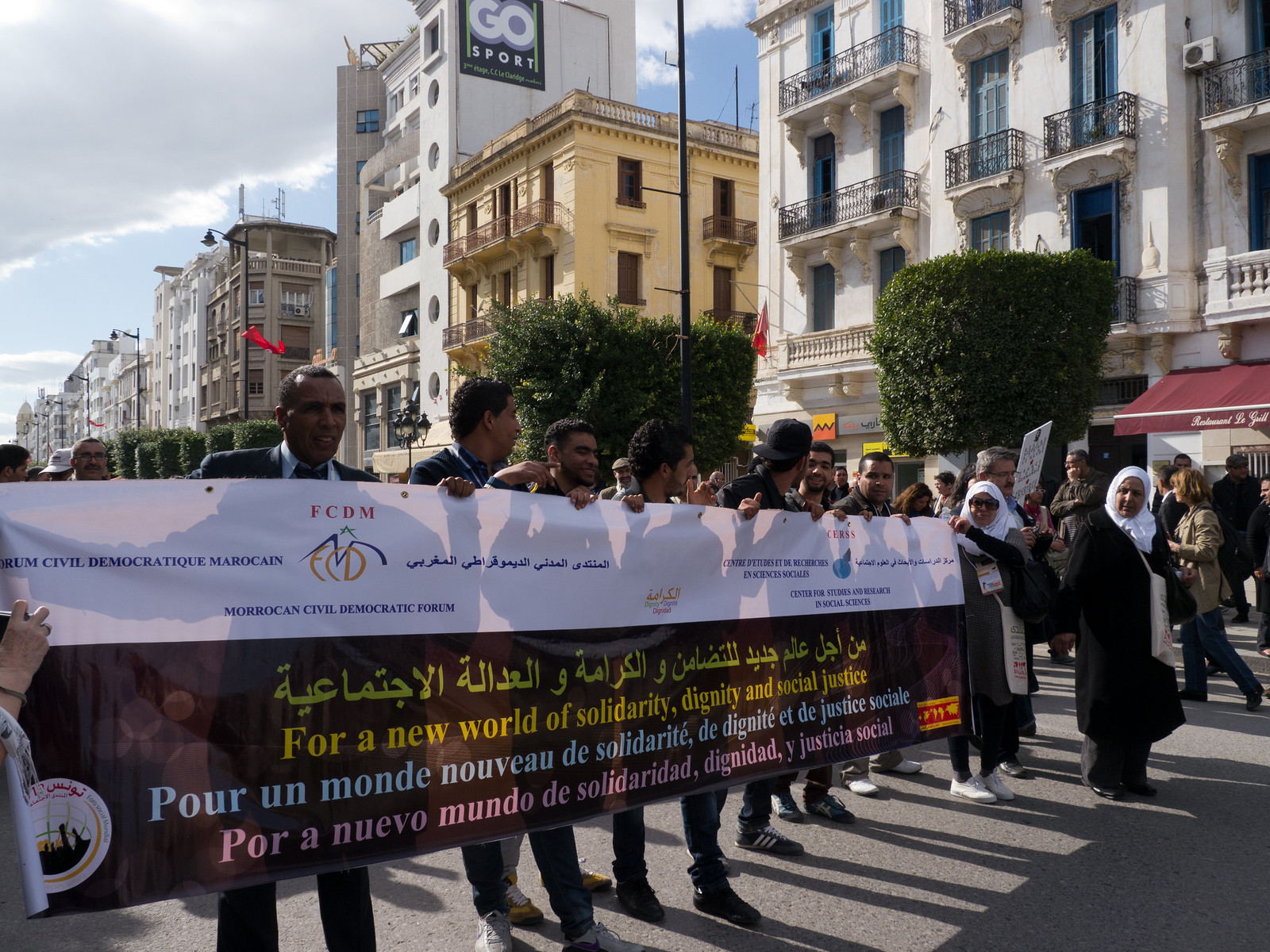The image captures a vibrant street protest or parade, prominently featuring a large, diverse crowd centered around a sign advocating for "a new world of solidarity, dignity, and social justice." The sign, white at the top and black at the bottom, is inscribed in multiple languages, with Arabic at the top, followed by translations in English, French, and Spanish. Above the crowd, a banner reads "FCDM, Moroccan Civil Democratic Forum," indicating a possible Moroccan origin of the participants.

The crowd, well-dressed and comprising individuals who appear to be of Middle Eastern or North African descent, occupies the middle of an all-grey street. Surrounding the scene are old, well-maintained buildings suggesting a significant urban center, potentially in the Middle East, North Africa, or even a European country. To the right, some women are dressed in black, burqa-like outfits with white headwrappings, blending with the mix of bystanders and pedestrians, some of whom seem engaged in their daily routines such as shopping.

In the background, large green bushes and streetlights flank the buildings, adding depth to the outdoor setting. The sky above is partly cloudy with patches of blue, indicating a mid-day context for this political demonstration. Colors in the scene include grey, white, light blue, brown, tan, yellow, purple, pink, maroon, enhancing the image's vividness and emphasizing its dynamic atmosphere.